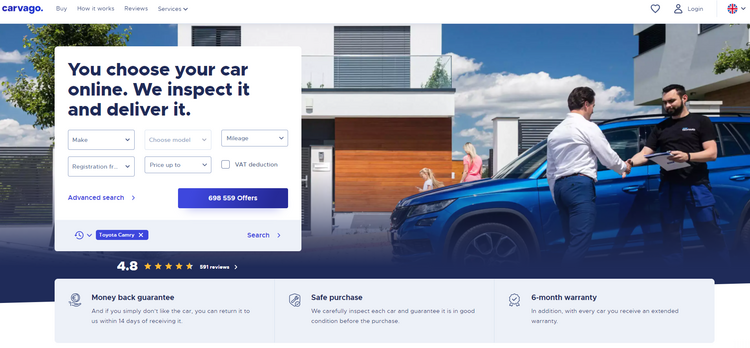The screenshot depicts the homepage of Carvago, showcasing its landing page. The top-left corner features the Carvago logo set against a white banner. Dominating the page is a large splash image of two men shaking hands, symbolizing a successful transaction. The prominent tagline reads, "You choose your car online. We inspect it and deliver it," highlighting the company's service promise. Below this, there is a set of form fields designed for users to fill out to receive offers. At the bottom of the image, a gray rectangular banner spans the width of the page, emphasizing key selling points: "Money-back guarantee," "Safe purchase," and "Six months warranty." Additionally, the top-right corner includes utility icons such as a heart for favoriting items, a login button, and a country selector.